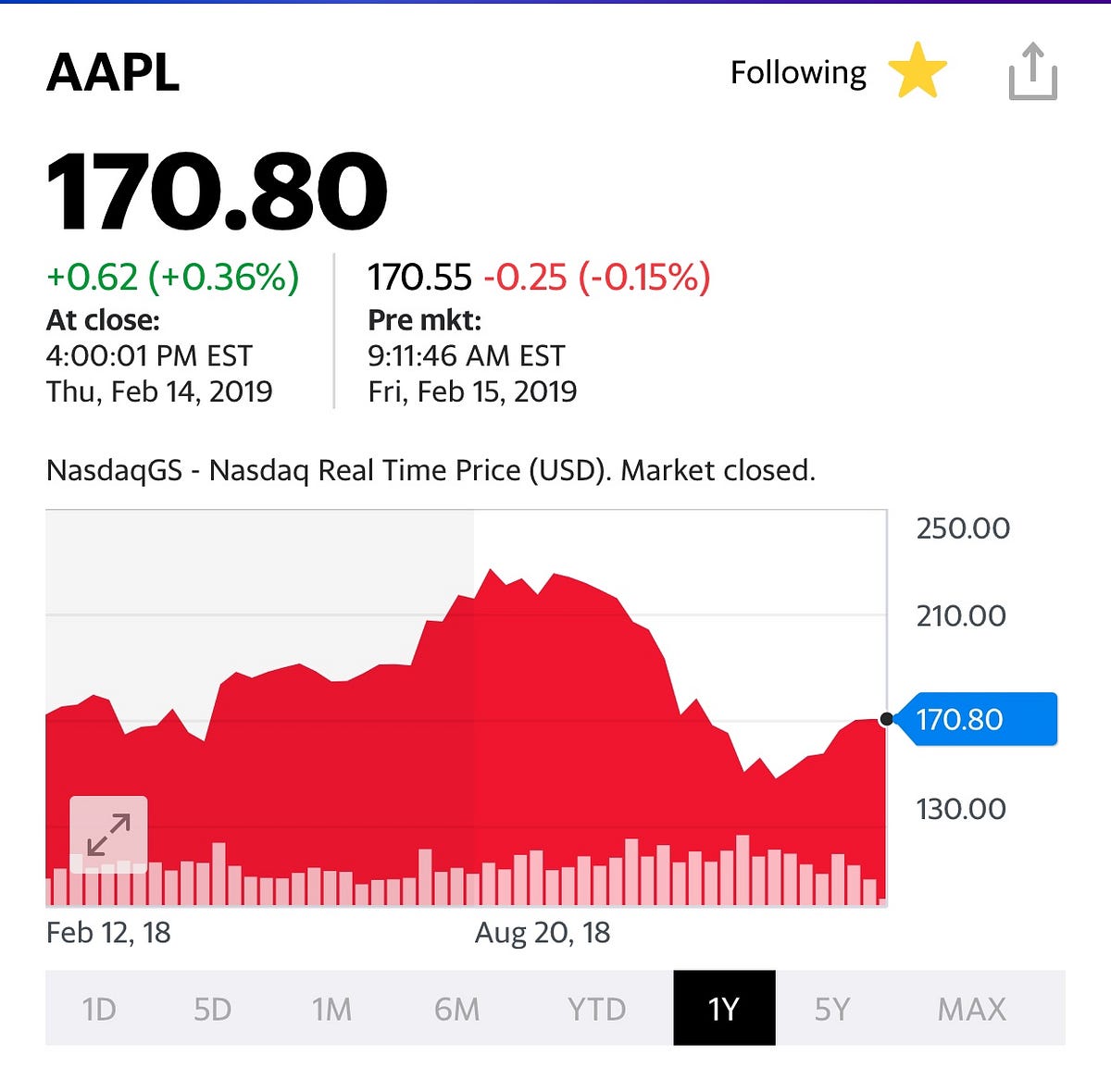The image displays detailed stock information for Apple Inc. (AAPL). In the top left corner, "AAPL" is prominently displayed, identifying the stock's ticker symbol. The top right corner features the word "Following" with a yellow star and an upwards-pointing arrow, indicating that this stock is being tracked closely.

The current stock price is shown as "$170.80," with a daily increase indicated by "+0.62 (+0.36%)." This price was recorded at market close at 4:00 PM or 1:00 PM Eastern Time on Thursday, February 14, 2019. Adjacent to this, the pre-market price is listed as "$170.55," reflecting a slight decrease of "-0.25 (-0.15%)" as of 9:11:46 AM Eastern Time on Friday, February 15, 2019.

Beneath the pricing information, a graph charts the stock's performance from February 12, 2018, to August 2018. The graph is rendered with red lines, illustrating the stock's fluctuations, marked by various peaks and valleys. Above the graph, the text "NASDAQ GS" and "NASDAQ real-time price. USD. Market closed." provides further context.

On the right side of the graph, a vertical axis lists price points ranging from $130.00 to $250.00, with the current price of $170.80 highlighted in blue. At the graph's bottom, a timeline navigation bar features options labeled "1D, 5D, 1M, 6M, YTD," with "1Y" highlighted to indicate the one-year view is currently active. Additional options "5Y" and "MAX" follow the highlighted section, allowing for expanded views of the stock's historical performance.